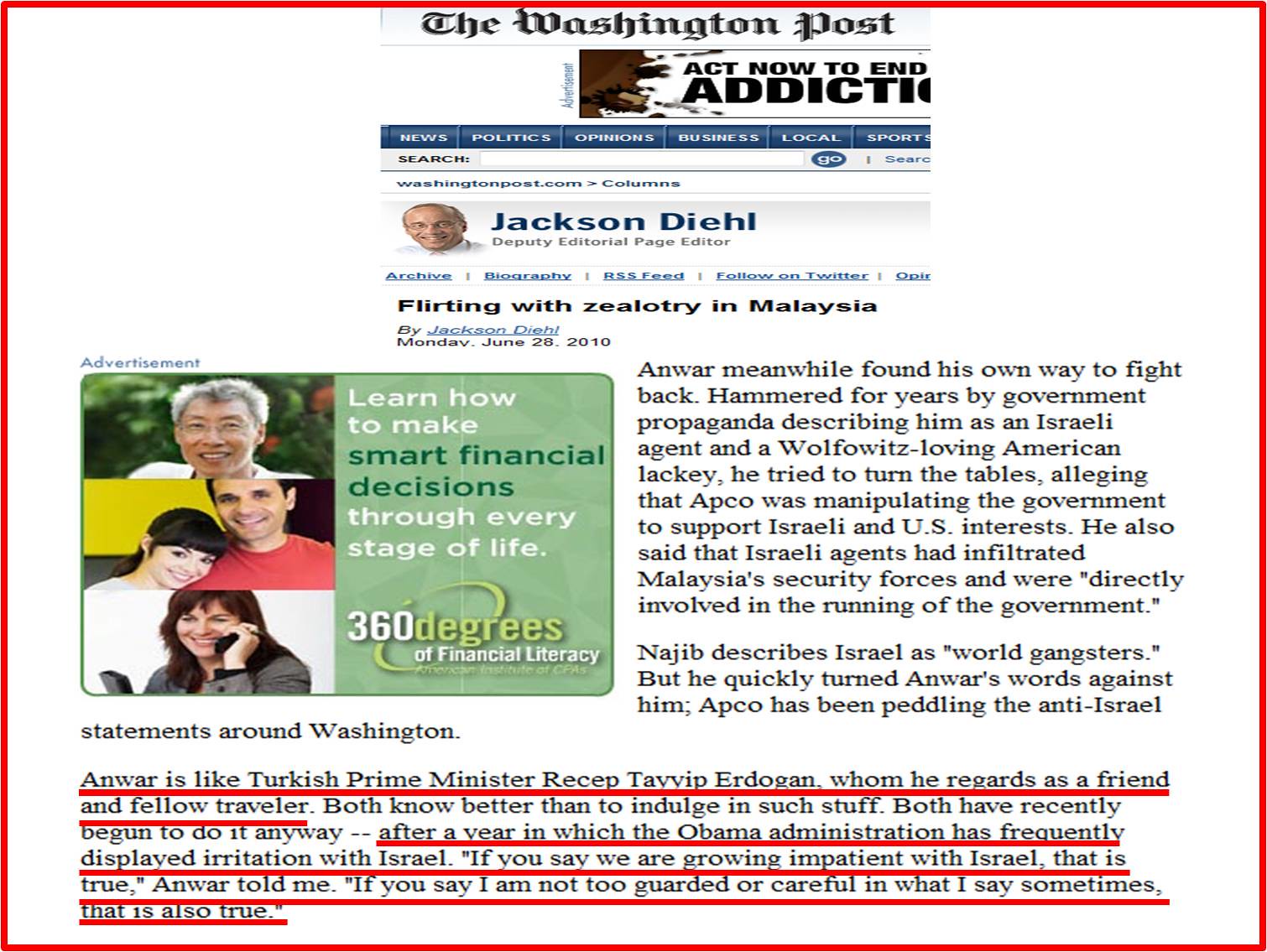The image depicts a web page from The Washington Post displaying an article written by Deputy Editorial Page Editor Jackson Diehl, titled "Flirting with Zealotry in Malaysia." The web page features a white background with black lettering, punctuated by various ads and menu bars. At the top, a prominent advertisement urges readers to "Act Now to End Addiction." Below this, the website's navigation menu includes categories such as News, Politics, Opinions, Business, Local Sports, and more.

The main focus is an article discussing Anwar, who has been criticized for years by government propaganda labeling him as an Israeli agent and a Wolfowitz-loving American lackey. In retaliation, Anwar claims that APCO is manipulating the Malaysian government to back Israeli and U.S. interests, even alleging that Israeli agents have infiltrated the country's security forces. Najib, on the other hand, criticizes Israel as "world gangsters" and counters Anwar's statements. The article also draws comparisons between Anwar and Turkish Prime Minister Recep Tayyip Erdogan, noting both leaders have recently made controversial comments about Israel amidst growing impatience from the Obama administration.

Adjacent to the article on the right is an advertisement promoting financial literacy, featuring three sections of people's faces with a call to "Learn How to Make Smart Financial Decisions." The article itself is composed of two main paragraphs and a critical, almost fully underlined section at the bottom, which spans about five to six lines. The entire layout is framed by a thin red border, emphasizing its visual structure.